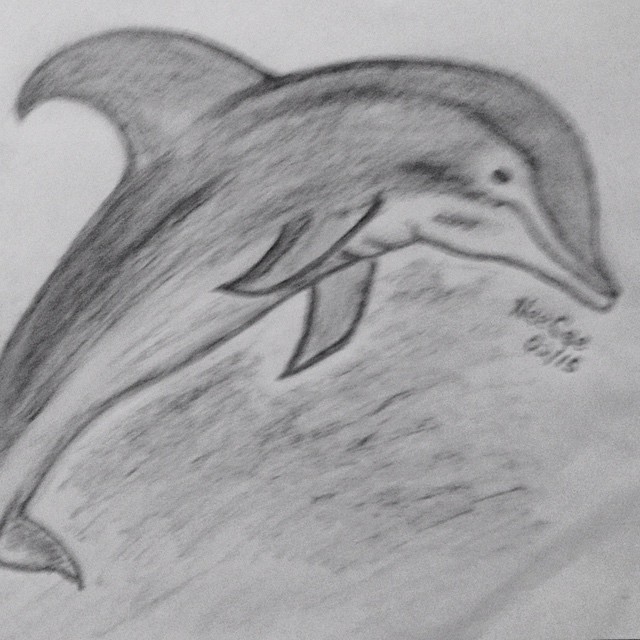This is a detailed pencil drawing of a bottlenose dolphin on white paper. The dolphin, captured in mid-jump out of the ocean, is portrayed from a side angle, leaping towards the right side of the paper. The shading work on the dolphin is exemplary, highlighting its smooth skin and anatomical details. Its prominent, tall dorsal fin and the smaller side fins (or flippers) are both well-shaded, adding depth to the drawing. The dolphin's body exhibits little folds of skin, emphasizing the dynamic motion of bending as it leaps. Notably, the dolphin has a bottle-shaped nose and a distinctive dark eye. Below the dolphin's nose, there’s text that reads “Knee Cage, 9-15," accompanied by the artist's signature, though the signature is blurred and not entirely legible. The artist has skillfully rendered the dolphin, giving it a lifelike appearance despite the pencil medium.